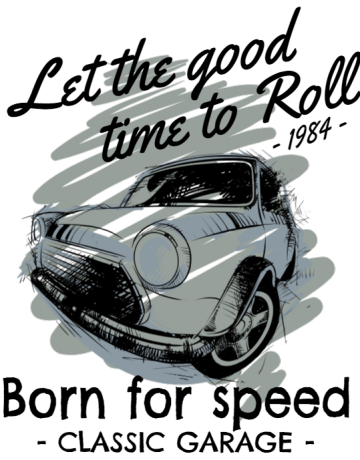The image is a digitally created black, white, and grey poster featuring a stylized sketch of a car. The car is positioned at a diagonal angle, prominently displaying the front, including one headlight, the grill, and the left front tire turned to the right. The windshield and interior details are blacked out, adding a mysterious touch to the sketch. A grey, squiggly ink mark overlays parts of the car, resembling the carefree coloring of a child.

At the top of the image, in a combination of black text and script, the caption reads "Let the good time roll, 1984." Below the car, in a different black font, is the phrase "Born for speed," followed by "Classic Garage" in capital letters at the bottom. The overall aesthetic is minimalistic, defined by varying shades of grey and a white background.